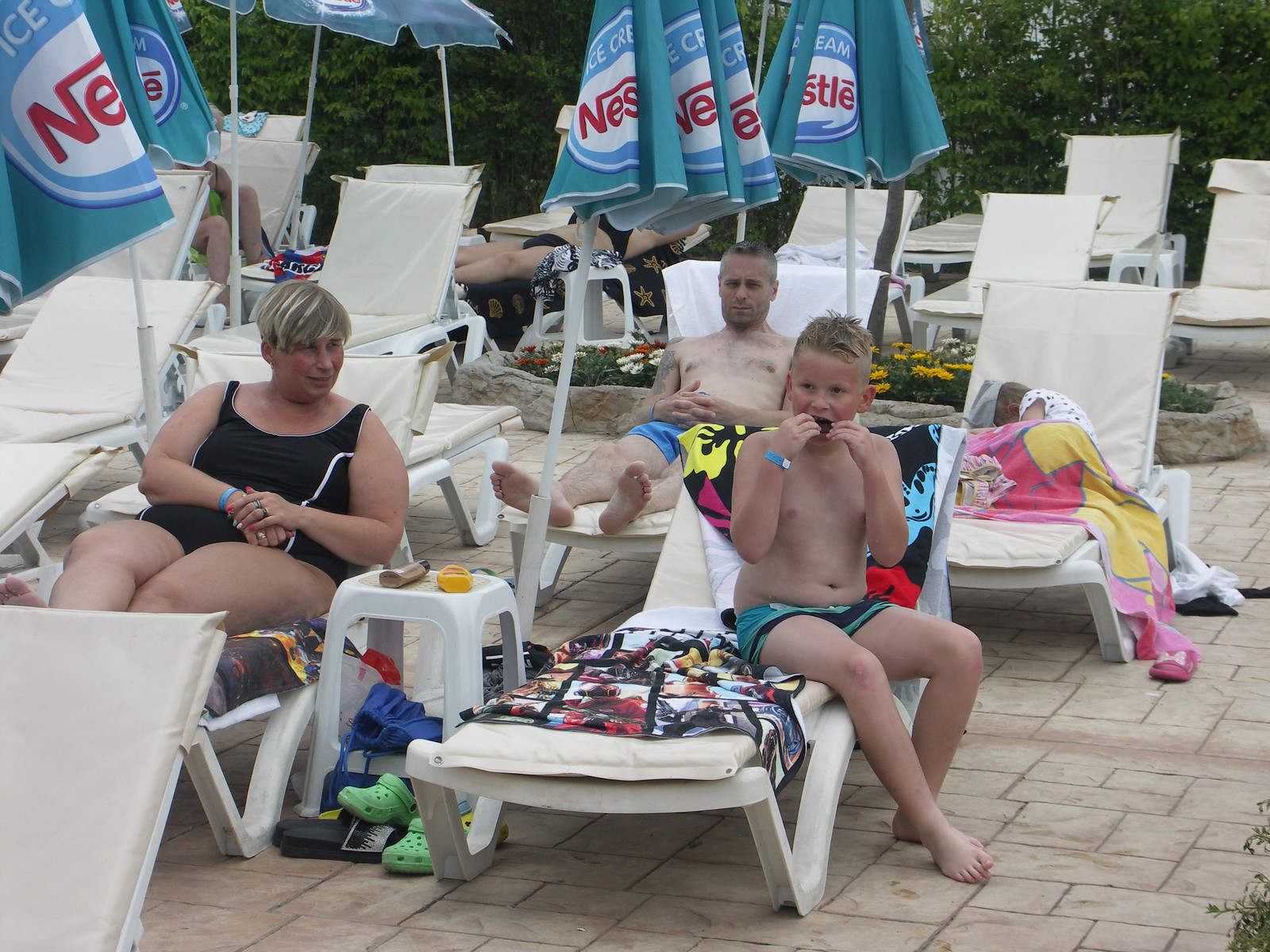In this horizontal rectangular image, a tranquil resort-like scene unfolds with an array of white lounge chairs neatly arranged on a tiled surface, likely near a swimming pool that remains out of frame. These chairs are shaded by blue Nestle umbrellas, identifiable by their white circles and red "Nestle" lettering. Scattered across the scene are varied-colored beach towels and personal belongings, hinting at recent or anticipated use. The foreground prominently features a young boy with light hair, wearing blue shorts and a matching wristband, seated on a lounge chair while eating a snack, his legs casually draped over the side. Beside him is a woman with very short, blond-streaked hair resembling a man's haircut, dressed in a one-piece black bathing suit, also wearing a blue wristband, and sitting on a towel on her lounge chair. A bit further back, lounging under the shade, is an older, very pale man with short hair in blue shorts, seemingly relaxing on his chair. Nearby, a small table holds items like a bottle, possibly flippers, and a pile of shoes. The backdrop includes lush trees, enhancing the serene ambiance of this partly occupied lounging area, with sunlight casting gentle shadows across the brick-tiled patio.